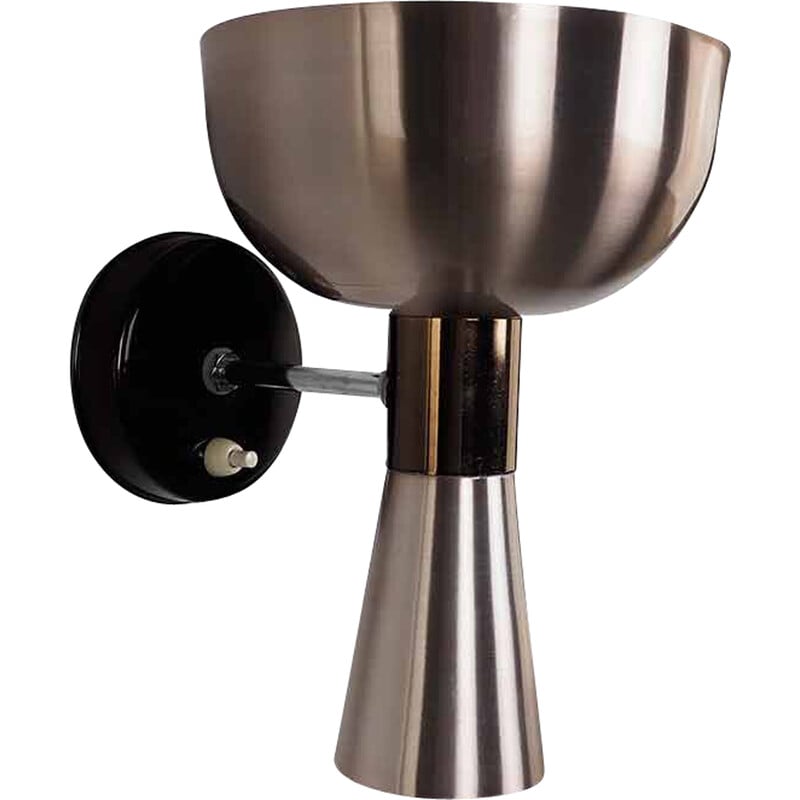This image depicts a close-up of a wall-mounted lamp featuring a sophisticated, multi-textured design. The lamp's main body resembles a large, brushed chrome goblet, characterized by a wide, rounded top that narrows into a thinner, conical-shaped bottom. This chrome structure is anchored to the wall by a gold-toned attachment, which gives the fixture an elegant contrast. The lamp is supported by a cylindrical black plastic wall mount, which has a distinctively modern aesthetic. This wall mount includes a prominent silver push-button switch located at the bottom, enhancing the lamp's functionality. The backdrop of the image is white, which highlights the sleek and metallic components of the lamp.